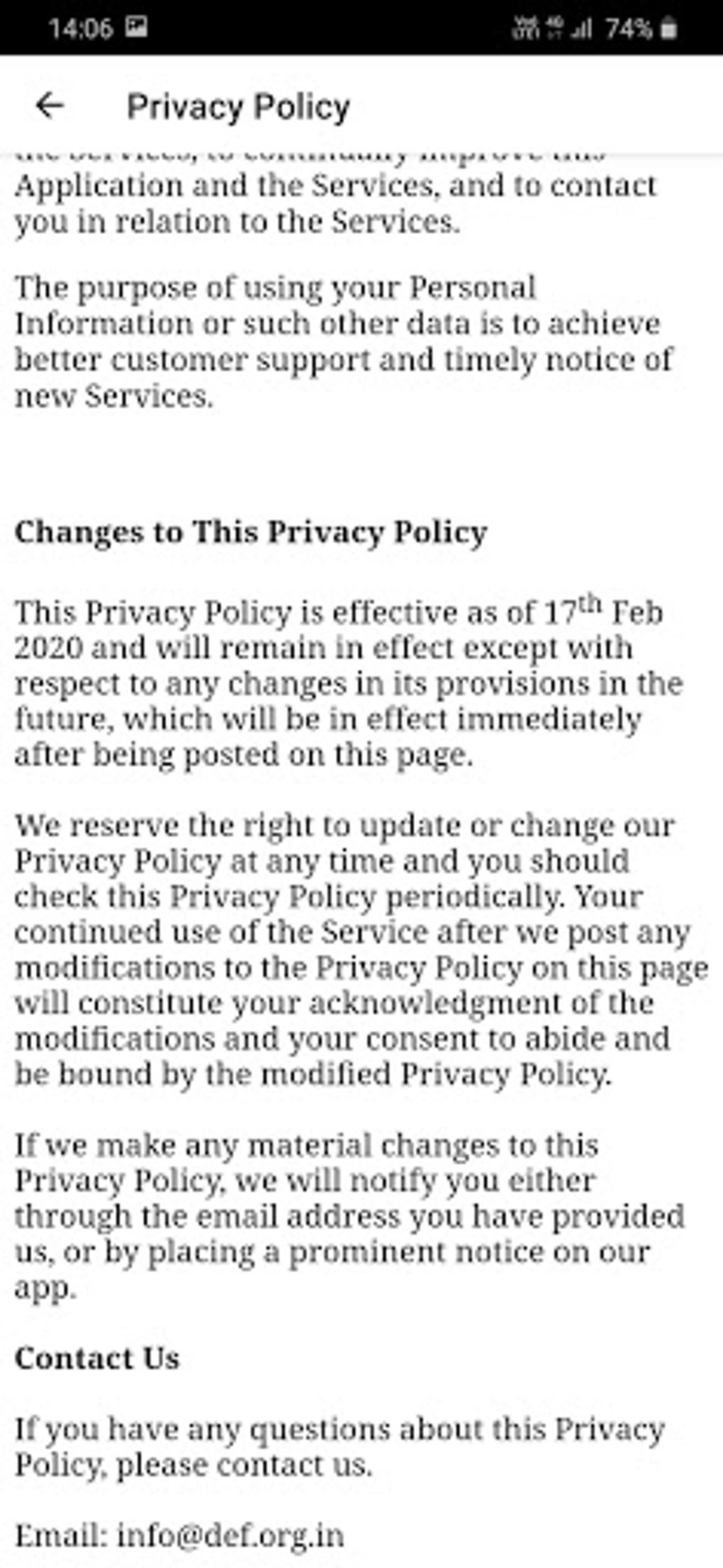In this screenshot, the top left corner displays the current time, while the top right corner shows the network signal bars, battery percentage, and a Voice over LTE (VoLTE) icon. Central to the image is a section of text detailing aspects of a privacy policy. The text elaborates on the application and the services provided, emphasizing the intention to use personal information to enhance customer support and notify users about new services in a timely manner. It also outlines the policy for changes, stating that the privacy policy is effective from February 17, 2020, and will remain in effect immediately after being posted on the site. The policy reserves the right to be updated or altered, advising users to periodically review the privacy policy for any changes.